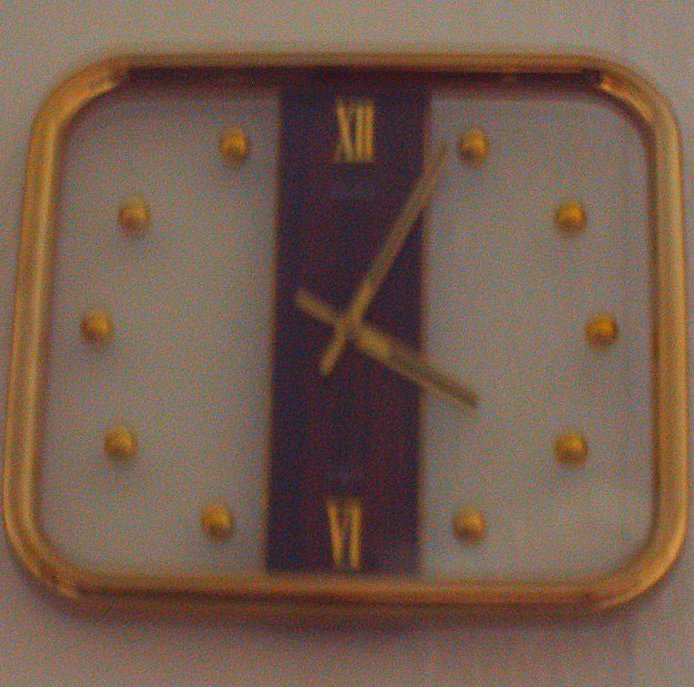This image depicts a slightly blurry rectangular wall clock set against a beige-colored wall. The clock features a clear, see-through face, with gold-toned minute and hour hands. It indicates the time as exactly 4:00. At the 12 o'clock and 6 o'clock positions, Roman numerals are displayed, while the positions of the other numbers are marked by round, ball-like indicators. The outer frame of the clock appears to be a tubular gold structure. Additionally, a brown line runs vertically through the clock, connecting the 12 and 6 positions, further dividing the transparent clock face. Notably, there is no visible brand name on the clock.